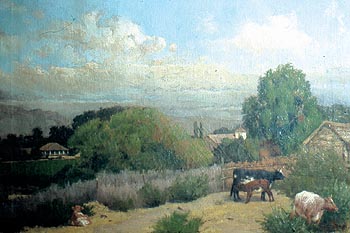This artwork is a detailed painting or watercolor of a serene countryside scene. Predominantly featuring a blue sky with white, moderately cloudy patches, the upper right corner is the brightest, possibly illuminated by the sun behind the clouds. The painting is filled with lush greenery, including dense groves of trees primarily on the right, and hints of rough foliage and grass scattered throughout.

In the lower right corner, three animals are depicted: a black and white cow, a brown and white calf, and another cow of lighter shade. One of the cows appears to be resting. Central to the composition are two figures, possibly people, adding a human element to the natural setting.

The scene captures a farmyard with notable elements such as a T-shaped or turret-roofed building, reminiscent of an Italian style, partially obscured by trees and foliage. There is a fence and barn situated amidst this landscape. Rocks or earthy brown elements are apparent near the bottom left.

The primary colors conveyed are white, blue, green, brown, and touches of black, creating a cohesive farmland panorama set against a backdrop of distant mountains. The artwork provides a tranquil snapshot of rural life, with no text or numbers present to distract from its visual narrative.